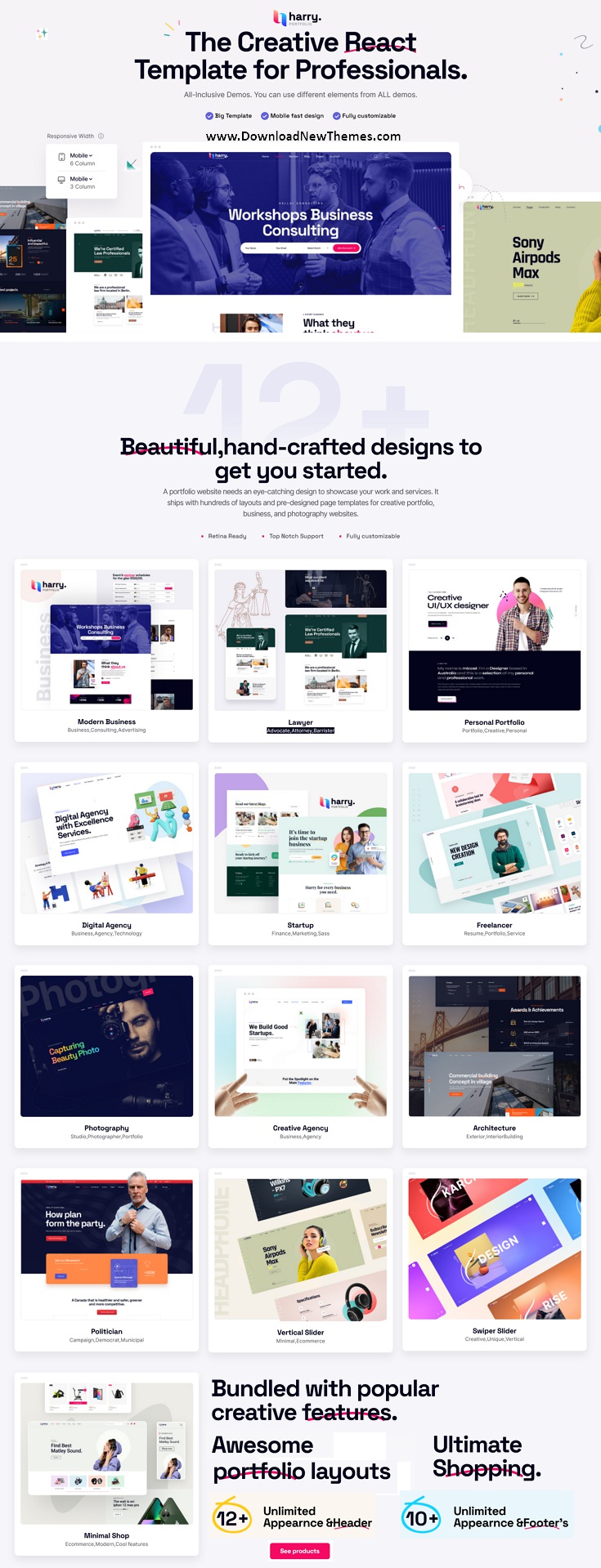The image showcases a vertically-oriented app or website interface with a light gray background, approximately three times as high as it is wide. At the top, centered in bold black text, is the title "Creative React Template for Professionals." Beneath this title, there are three lines of text too small to be legible.

Further down, there is a banner section divided into three segments. The left and right segments each occupy approximately 20% of the width, while a central blue segment takes up about 30%. The central segment features an image of four individuals, two on the left and two on the right, engaged in conversation from the waist up. The image is overlaid with white text that reads "Workshops, Business Consulting."

Continuing downward, centered black text states "Beautiful handcrafted designs to get you started." Below this, another four lines of small, unreadable text appear.

The lower portion of the interface consists of a grid displaying various designs, arranged in a 3x4 format. Additionally, there is one extra design placed to the left of the grid, collectively showcasing a total of thirteen different design options.